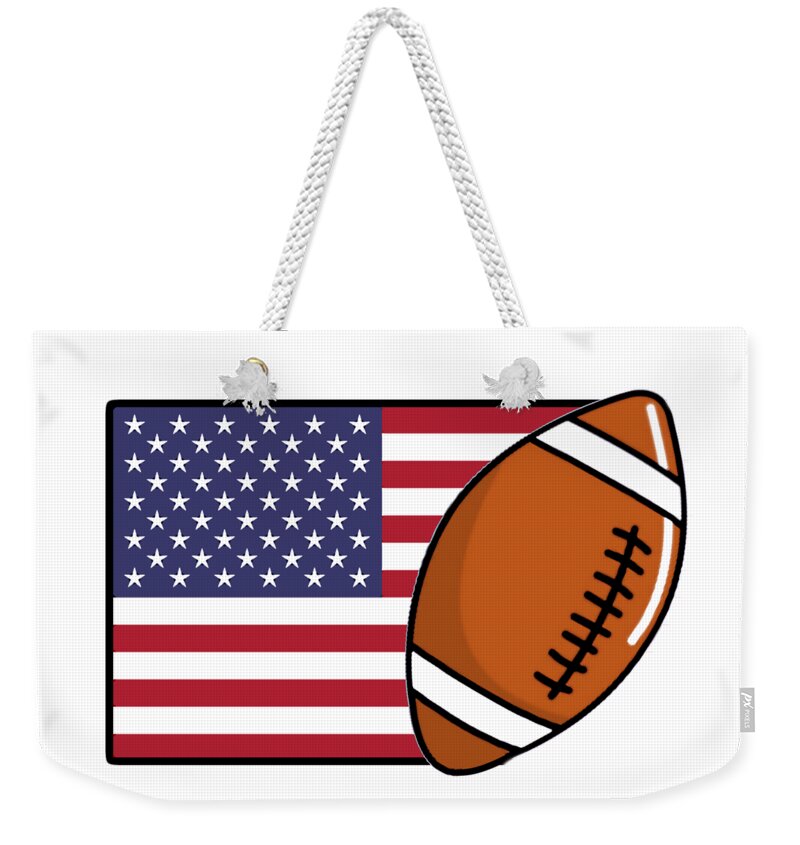This photograph captures a white canvas tote bag set against a plain white background. The tote bag, designed with a sturdy braided rope handle threaded through silver grommets and secured with knots, features a prominent design of an American flag. The flag, covering a substantial portion of the bag's surface, displays its blue field of white stars in the top left corner, with the red and white stripes extended across. Overlaying the right-hand side of the flag at an angle is a detailed image of a large, brown football characterized by white stripes and black laces. A small black tag is visible in the bottom right corner of the bag. The bag's medium size suggests it could be practical for carrying essentials to a football game, the beach, or the pool.